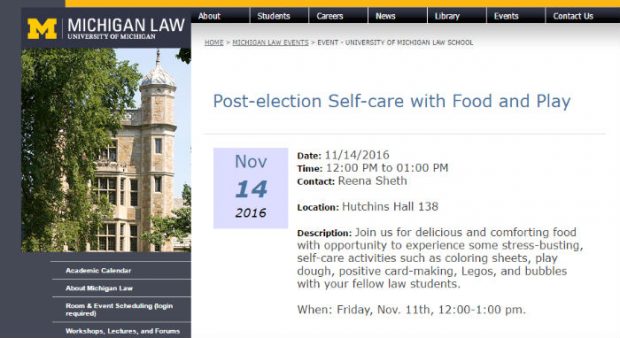Join us at the University of Michigan Law School on Monday, November 14, 2016, from 12:00 PM to 1:00 PM for an event focused on post-election self-care, held in Hutchins Hall 138. This session offers a unique opportunity for law students to unwind and de-stress with delicious and comforting food, along with various self-care activities. Engage in stress-busting tips and techniques, including positive card-making, playing with Legos, blowing bubbles, and other playful activities alongside your fellow peers. Don’t miss out on this chance to relax and rejuvenate during a busy academic semester. Event details: November 14, 2016, from 12:00 PM to 1:00 PM, Hutchins Hall 138.